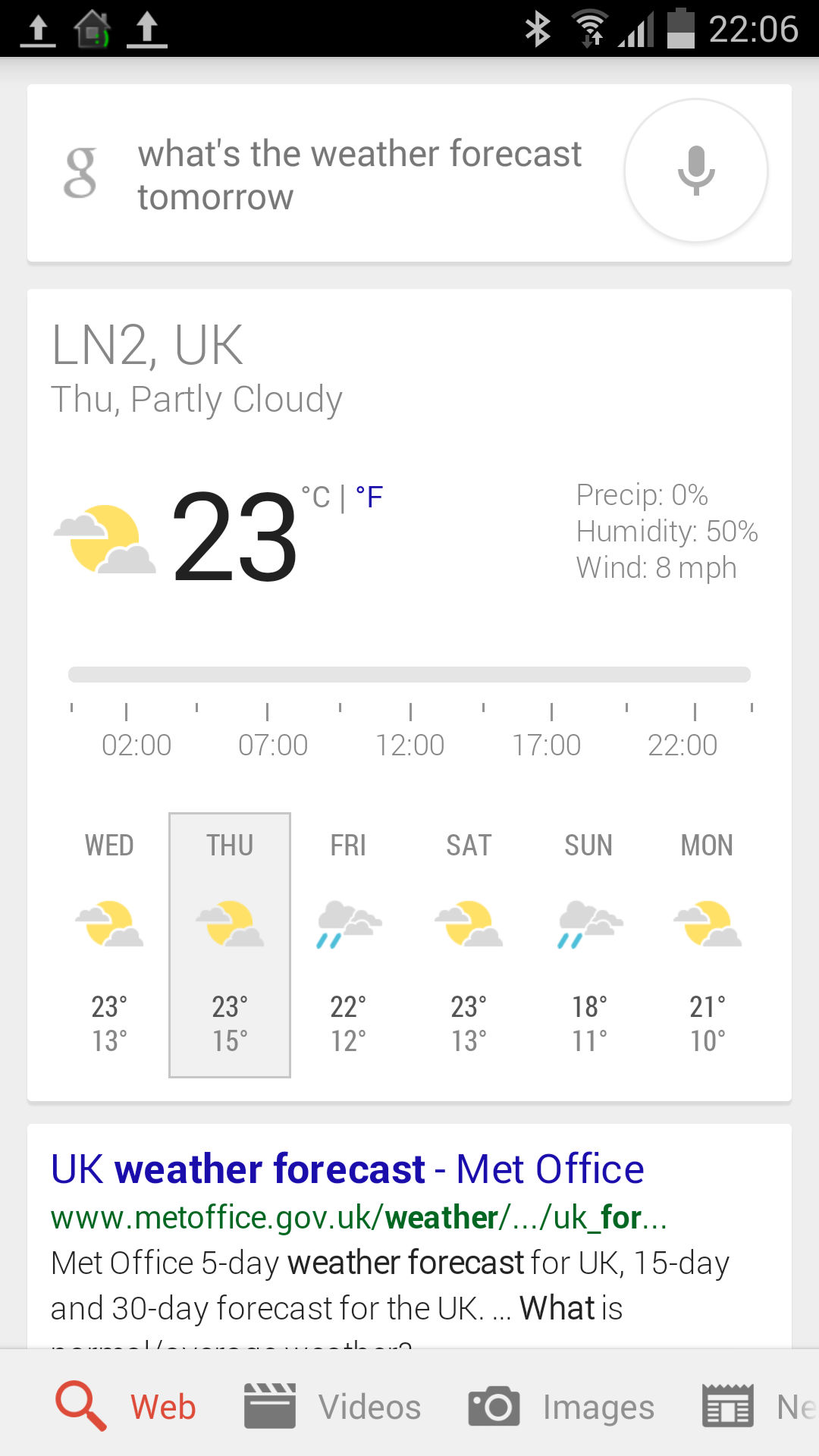This image is a screenshot of the Google App Browser on an Android device. At the very top of the screen, a notification bar displays various icons, including those for Bluetooth, Wi-Fi, signal strength, battery status, and the time, located in the top right corner. Directly below this notification bar is the prominent Google icon, occupying a central position.

Beneath the Google icon is a large microphone icon, indicating the option for voice search. The main focus of the screen is a sizable white rectangular search bar that spans much of the display. Inside this bar is text indicating the location "LN2, UK," and a weather forecast for Thursday, noting "Partly Cloudy" with a temperature of 23 degrees Celsius.

To the right of this information, additional weather details are provided: a "Press C" reading at 0%, humidity at 50%, and wind speed at 8 MPH. The entire layout is cleanly designed, making the weather information clearly accessible.